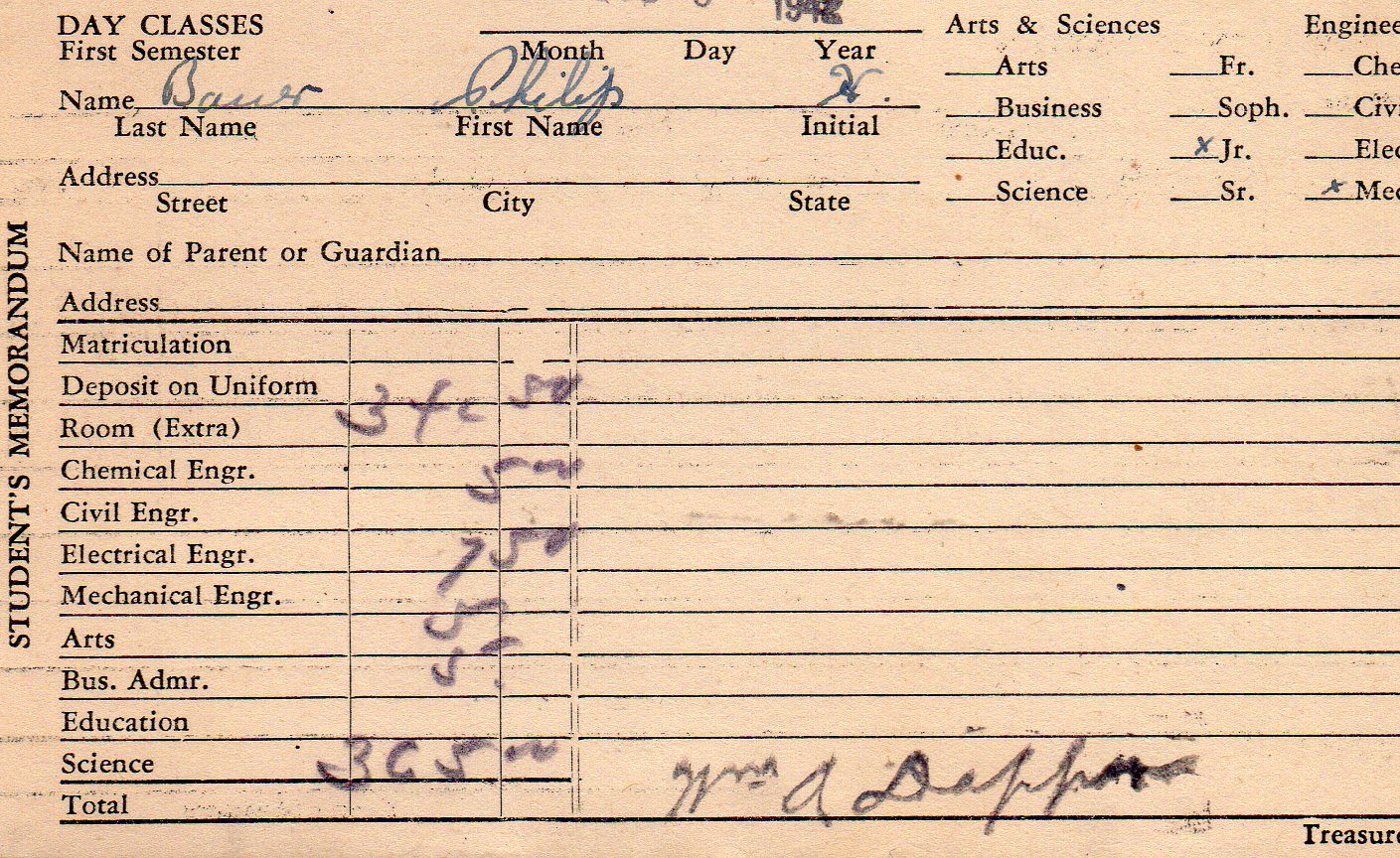The image depicts an old, yellowed student memorandum card, evocative of the 1940s, likely mimeographed. The card features both printed and handwritten elements. At the top left, it reads "Student's Memorandum," with sections for "Day Classes" and "First Semester." It includes blank spaces for filling in the student's name (with "Bauer, Philip" partially visible), address, city, state, and the name of a parent or guardian, though these fields remain empty. The card has options to check off for fields like Arts, Business, Education, Science, and the student's year (freshman, sophomore, junior, senior), with "junior" checked off. Different sections outline potential costs, such as Matriculation, Deposit on Uniform, and Room, alongside charges specific to majors like Arts, Business Administration, Electrical Engineering, Chemical Engineering, Civil Engineering, Education, and Science. Handwritten numbers are present in some fields, indicating the amounts owed, with a total cost noted as $365. There is a signature at the bottom right, suggesting the form's completion, and an overall impression that the room charge might have been the most costly item. The document's aged appearance and specific reference to 1940s educational terms enhance its historical authenticity.